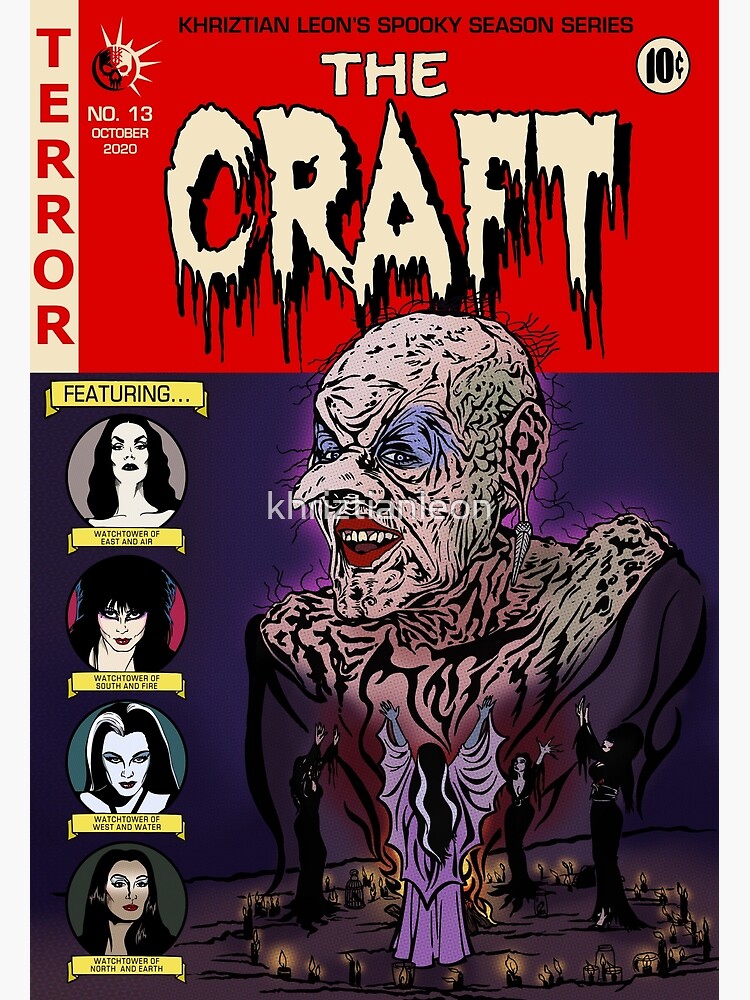The image is a vibrant and detailed poster for a television series titled "Christian Leon's Spooky Season Series," with the words “Christian” stylized as "K-H-R-I-Z-T-I-A-N" written in black text on a striking red background at the top. Prominently, the title "The Craft" is rendered in white letters that appear to be dripping black wax. The poster also features details such as "10 cents" in the top right corner and "Terror" in red, running vertically on the left margin. It is marked as issue "No. 13, October 2020."

A central figure stands out—a monstrous creature with a white and black face adorned with stripes and swirls, bright blue eyes, red lips, and a sharply pointed nose. Its massive shoulders dominate the bottom portion of the poster, with smaller figures encircling it in a manner that suggests worship or ritualistic praise. Among these figures are iconic characters like Vampira, Elvira, Lily Munster, and Morticia Addams, positioned around the larger creature, each recognizable despite the tiny, unreadable yellow labels beneath them. Purple, red, white, and black hues create a spooky yet captivating atmosphere throughout the poster.

Additionally, there is a watermark, "Christian Leon," across a witch drawn prominently in the center, potentially associated with the movie "The Witches." The overall design contains elements reminiscent of gothic horror art, blending classic horror icons and mysterious ritualistic imagery, making it both eerie and intriguing.